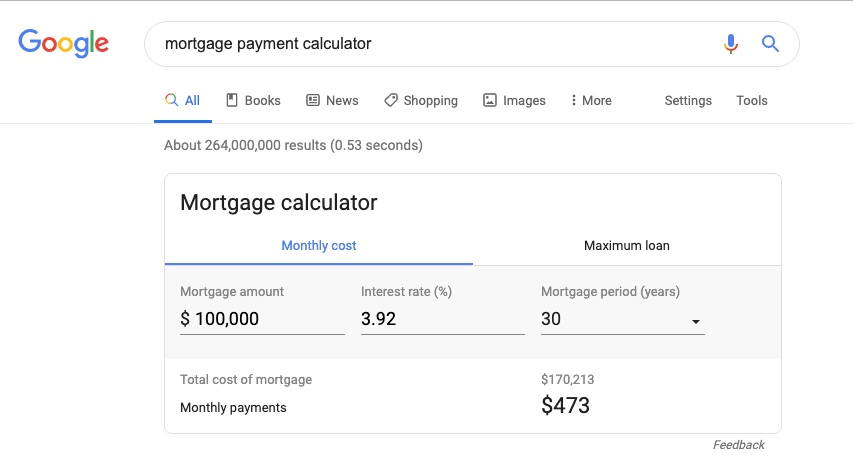This image is a screenshot of the Google website. In the upper left-hand corner, the iconic "Google" logo is prominently displayed. To the right of the Google logo, there's a search bar containing the query "mortgage payment calculator," alongside a microphone icon and a magnifying glass search icon.

Beneath the search bar, there are navigational tabs labeled "All," "Books," "News," "Shopping," "Images," "More," "Settings," and "Tools." The "All" tab is highlighted in blue and underlined, indicating it is the active option. Directly below these tabs, the search results display indicates approximately 264 million results were found in 0.53 seconds.

A box bordered by gray lines is prominently featured, and it contains a Google tool interface labeled "Mortgage Calculator" at the top left. This interface is divided into two sections: "Monthly cost" and "Maximum loan," with "Monthly cost" highlighted in blue and underlined.

Under the section "Monthly cost," several fields are visible:
- Mortgage amount: $100,000
- Interest rate: 3.92%
- Mortgage period (years): 30

At the bottom of this section, the total cost of the mortgage is summarized. It shows a total mortgage cost of $170,213, with monthly payments specified as $473.